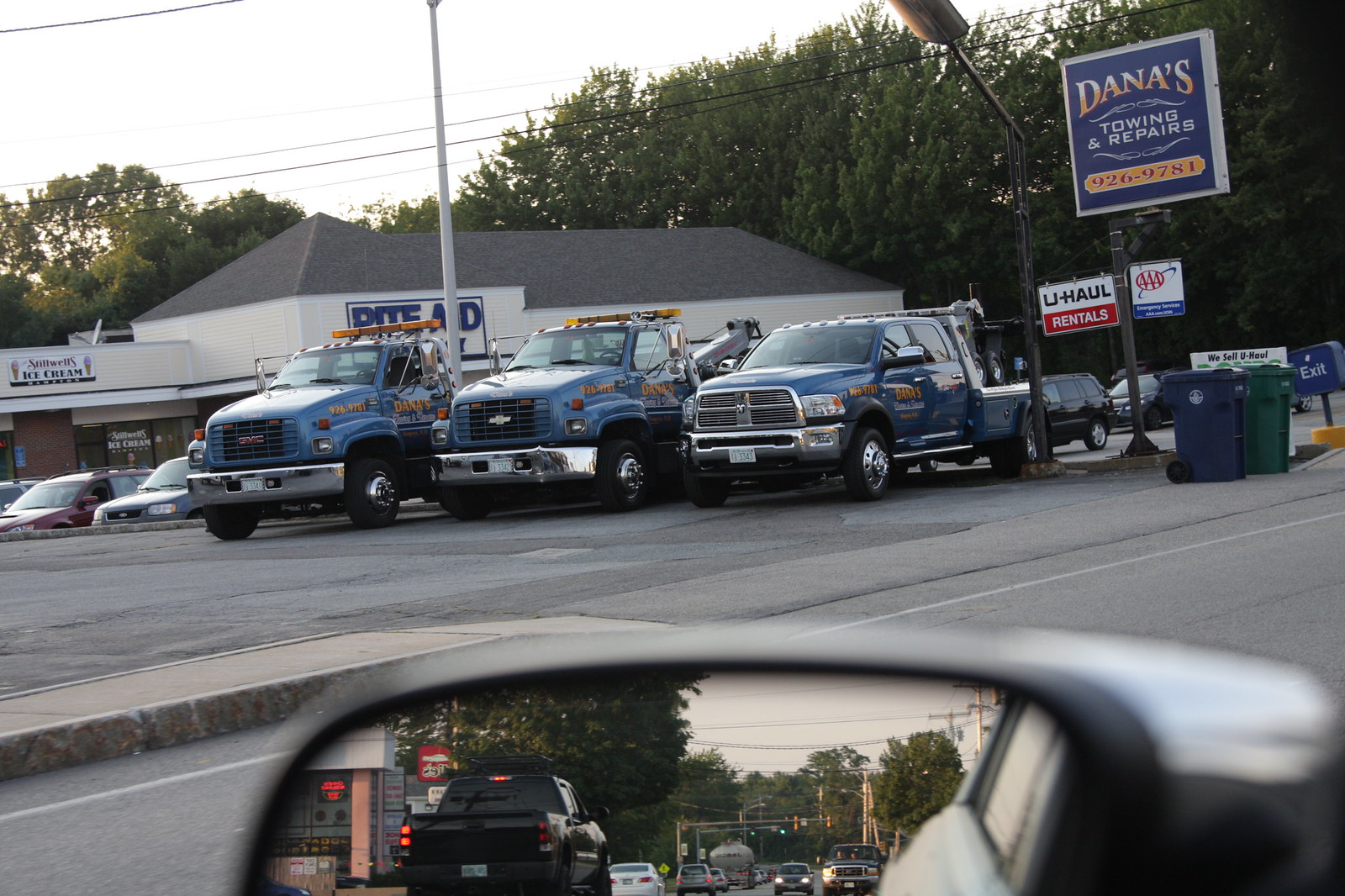The photograph captures a scene from inside a car parked in a lot, possibly at a shopping center. The lower part of the image is dominated by the reflection in a black rear-view mirror, showing a road with several cars and trucks behind, as well as a tree line against a grayish sky. Within the mirror, the photographer's partial reflection is also visible. The main view, however, shows a parking lot with three blue tow trucks equipped with yellow lights, all clearly marked with "Dana's Towing and Repairs," lined up horizontally in spaces. To the right, a significant sign atop the building promotes "Dana's Towing and Repairs," with a U-Haul logo beneath it. Behind these trucks, the white or tan building extends across the image, featuring a Rite Aid sign and another store sign that appears to mention ice cream. The entire area, including the asphalt lot, reflects a bustling, utilitarian atmosphere. Additionally, there are green and gray trash bins on the right side of the parking lot. The top of the image is framed by more sky and a tree line, completing the outdoor setting.